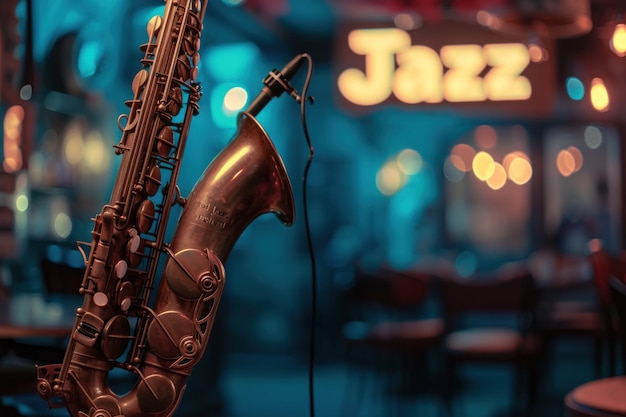This detailed image showcases a close-up view of a saxophone, meticulously drawn or captured, although the mouthpiece is absent, suggesting a zoomed-in perspective that omits the instrument's top part. Connected to the saxophone is a microphone or a recording device precisely mounted near the bell, with its cable trailing downwards. The background features an indeterminate, blurred blend of blue and green hues, with faint hints of possible chairs and softly blurred lights, contributing to a dreamy ambiance. In the upper right-hand corner, the word "Jazz" is inscribed in a hazy script, complementing the scene with an evocative, musical essence.